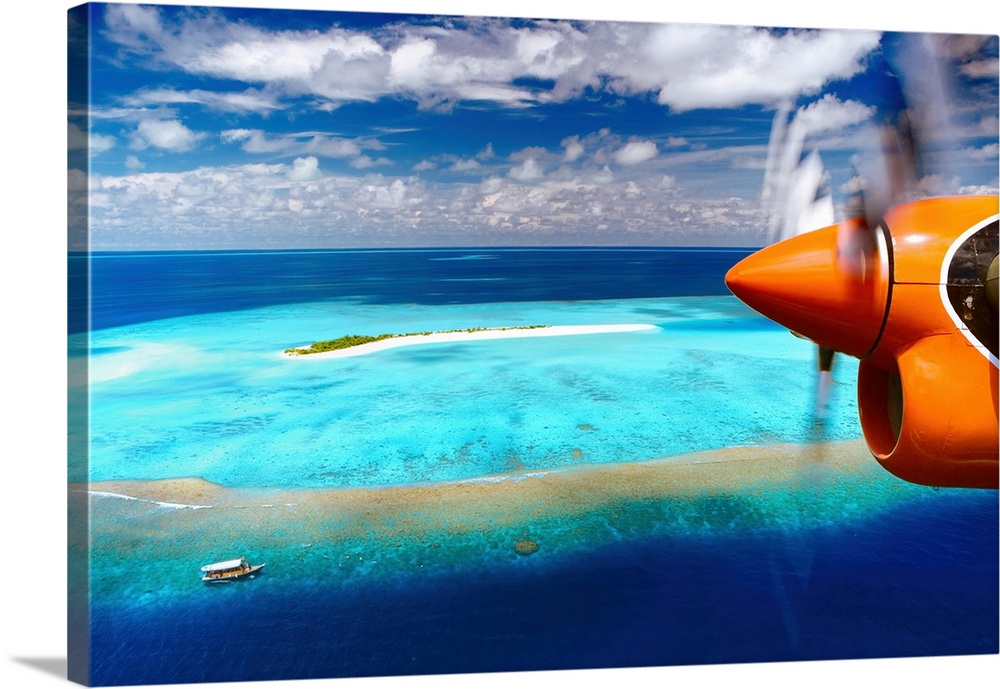This vibrant, photorealistic image, possibly mounted on a canvas, presents a stunning aerial view of a small, sandy island surrounded by a mesmerizing gradient of ocean colors – from deep blue to turquoise, highlighting a lighter blue circle of shallower water around the island, with a brown reef or cay encircling it. Central to the island is a small patch of greenery, while the sky above boasts a multitude of fluffy white clouds. In the lower left corner, just outside the sandbar reef edge, there is a boat. On the right side of the image, the nose and spinning propeller of an orange plane suggest that the photograph was captured from the plane itself, as it soars through the dynamic sky. The detailed layers and vibrant tones of the ocean and sky, along with the island's vegetated and sandy composition, generate a captivating visual experience.